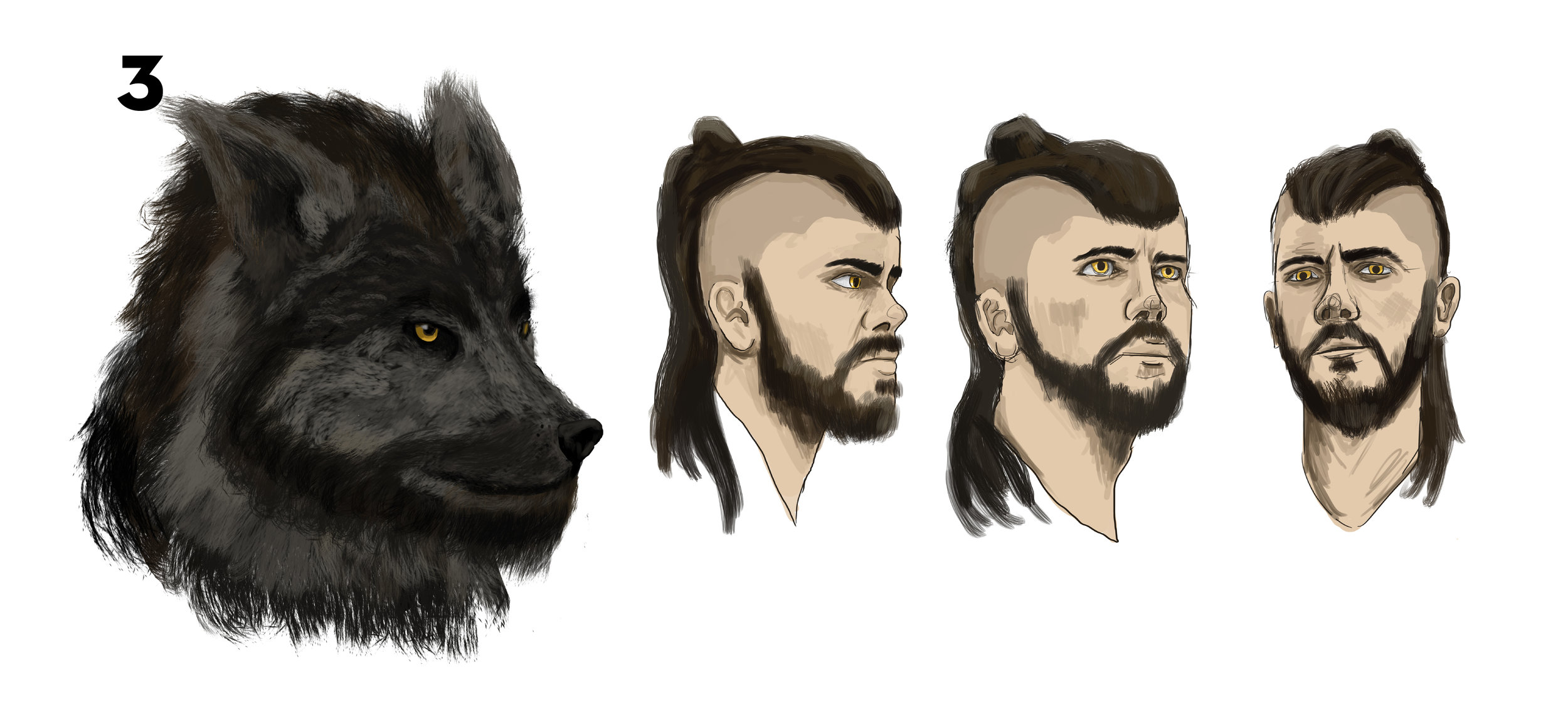The image showcases a transformative sketch centered around a black wolf character and a human male character, displayed against a white background. At the top left corner, the number "3" is visible, the only text in the image. On the left side of the image, the wolf's head is prominent, exhibiting a mix of gray and black fur, with piercing yellow eyes that convey a scary and intimidating look. The wolf appears almost anthropomorphic. On the right side of the image, there are three views of a Caucasian human male's head, each displaying different angles. He has long dark brown hair, styled in a way that could be gathered into a ponytail, and dark brown facial hair, including both a mustache and beard. The male character's eyes are also a striking yellow, akin to the wolf's, enhancing the transformative theme. His facial expression remains serious and solemn across the sketches, adding to the overall intensity of the design.